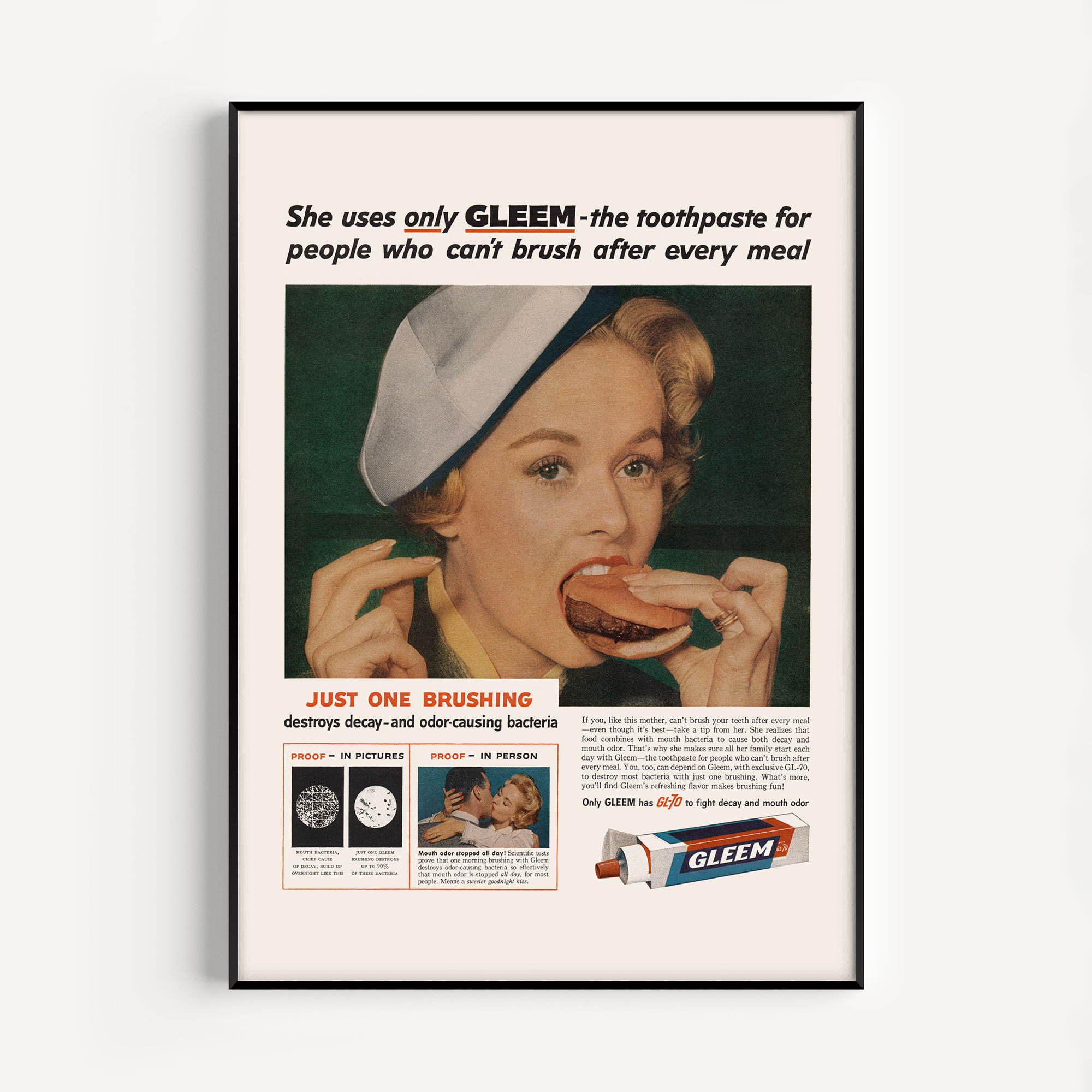This vintage advertisement for Gleam toothpaste features a striking black and white photograph framed in black. At the center of the image is a woman with short, curled reddish hair, adorned with a stylish beret on one side of her head. She is captured mid-bite, holding a large hamburger, her fingers on the other hand poised in a pinching gesture. The woman is dressed in a top with a visible yellow collar, adding a pop of color to the scene.

Above the image, bold black text proclaims, "She uses only Gleam, the toothpaste for people who can't brush after every meal." Below, an additional line promises, "Just one brushing destroys decay and odor-causing bacteria." 

The bottom of the advertisement is illustrated with a graphic representation of bacteria, emphasizing the toothpaste's efficacy. Adjacent to this, a romantic snapshot depicts a woman and a man kissing, highlighting the fresh breath benefit of using Gleam. Finally, to the right, a pristine white tube of Gleam toothpaste, encased in a stylish red, blue, and white box, is prominently displayed, completing the compelling visual narrative of this historic ad.